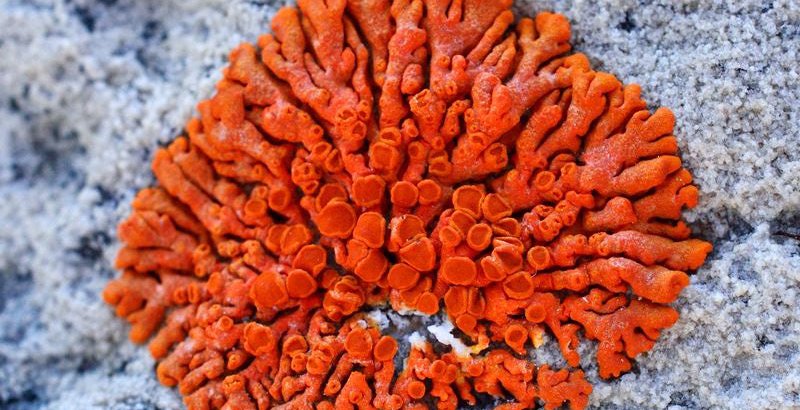The photograph showcases a microscopic close-up of an orange sea plant, with a somewhat round structure resembling a cluster of short, bubbly tubes or arm-like strands. These orange arms feature holes that are reminiscent of those in an octopus's limbs. The sea plant appears to be attached to a porous, gray surface, which serves as the background. The image, rectangular in shape and taken in landscape orientation, also has a snowy, white texture behind the main subject, possibly simulating a frosty or crystalline surface. The overall look suggests a detailed and complex structure, with the tubes fanning and branching out towards the edges, giving it a dynamic, organic appearance. The photograph's quality hints at a still frame from a video, adding to its intricate and vivid representation.